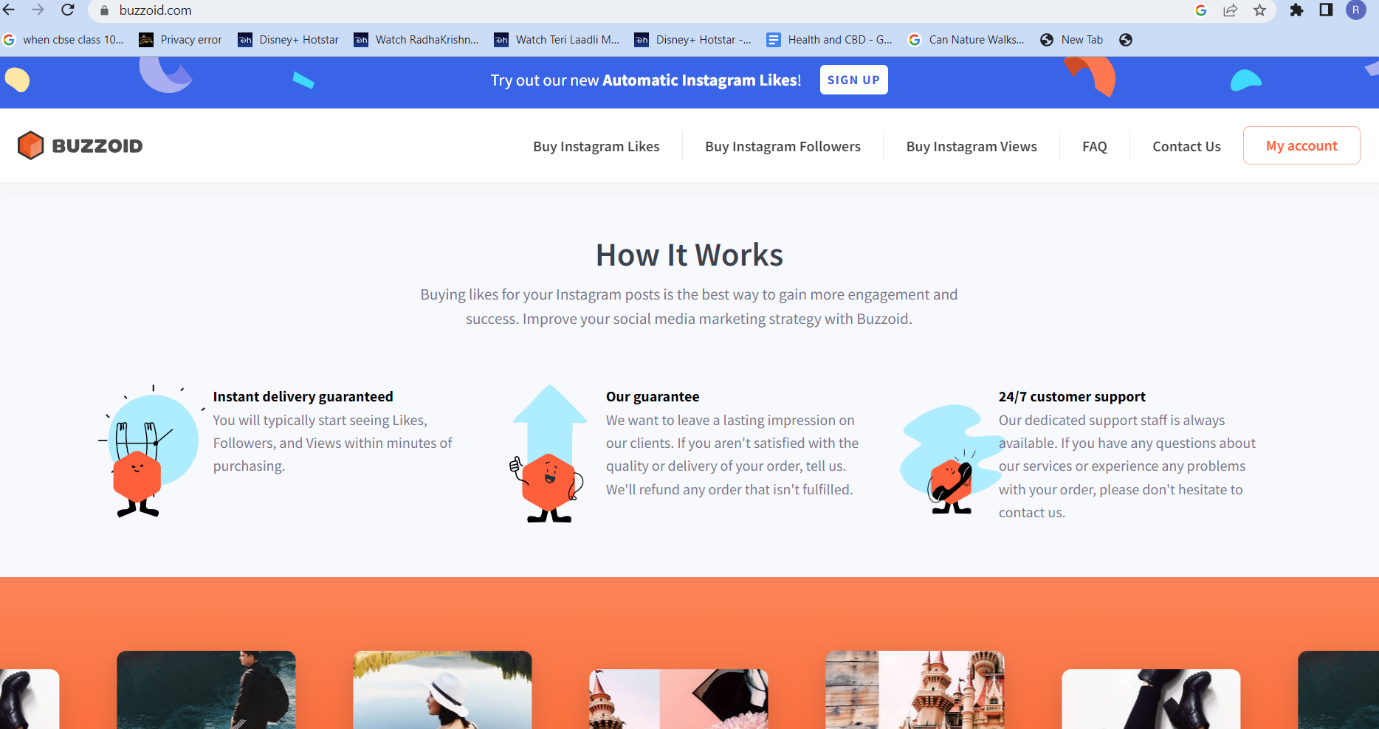The screenshot depicts a webpage from Buzzoid.com being viewed in Google Chrome. The browser tab lists several other open tabs, including: "CBSE Class 10," "Privacy Error," "Disney+ Hotstar," "Watch Radha Krishnan," "Watch Terry Leidy," "Disney+ Hotstar," "Health and CBD," "Can Nature Walks," and a new tab. 

Below the browser tabs is a pale blue navigation bar featuring multicolored shapes and white text that reads, "Try Our New Automatic Instagram Likes, Sign Up." 

The main content of the webpage is set against a white background and prominently showcases the Buzzoid branding with an orange square logo. Navigation options include links to "Buy Instagram Likes," "Buy Instagram Followers," "Buy Instagram Views," "FAQ," "Contact Us," and "My Account."

Further down, set on a pale gray background with black text, the site explains various features and benefits of its services under the heading "How It Works." The text claims that purchasing likes for Instagram posts is an effective way to increase engagement and success in social media marketing. Key points include:

- **Instant Delivery Guaranteed**: Users typically start seeing likes, followers, and views within minutes of making a purchase.
- **Our Guarantee**: Buzzoid promises satisfaction and offers refunds for orders that are not fulfilled.
- **24/7 Customer Support**: Dedicated support staff are always available to assist with any questions or issues related to the services provided.